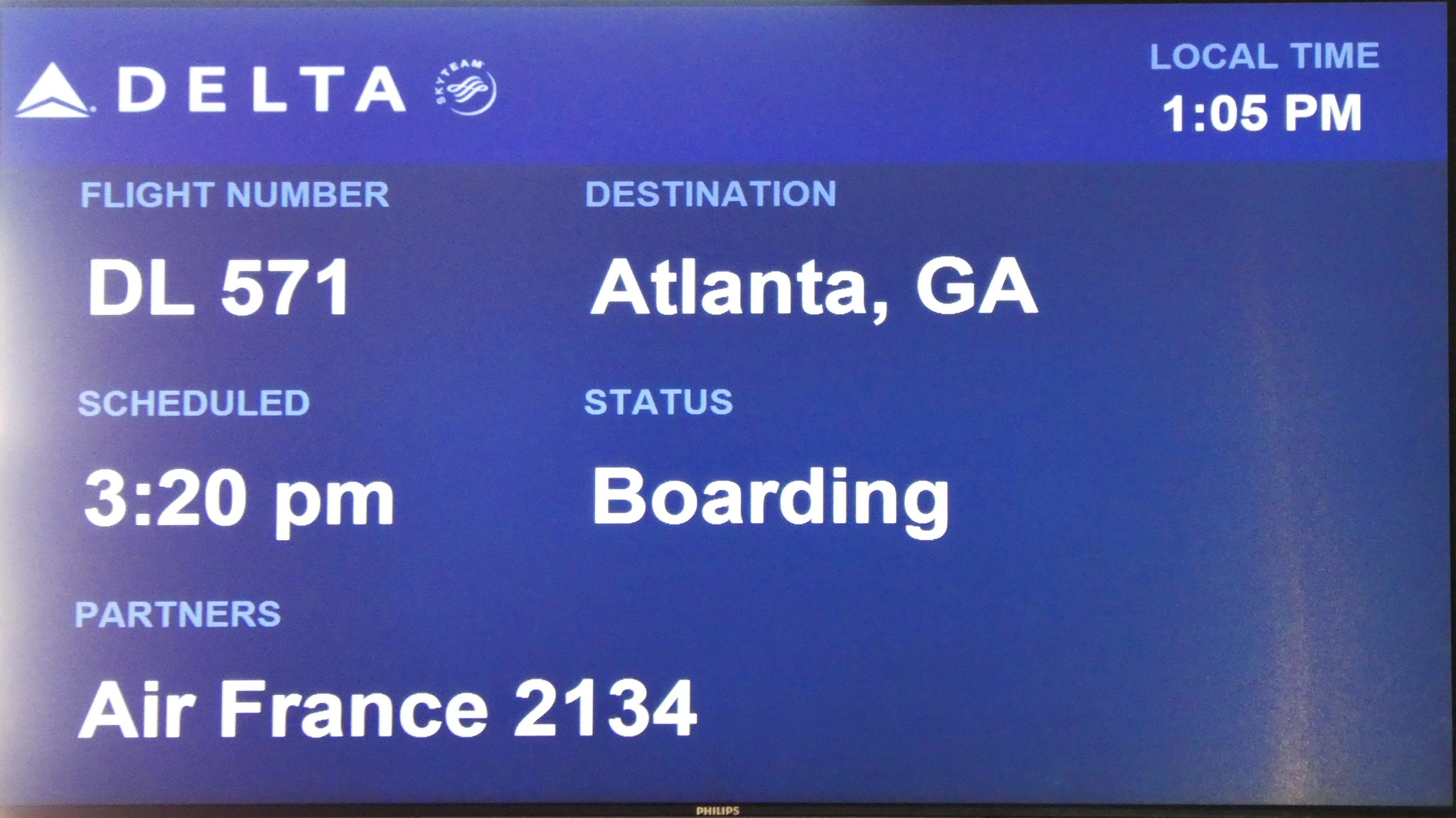The image displays a Delta Airlines flight information board at an airport. The screen features a blue background that transitions from light blue at the top to dark blue at the bottom. In the upper left corner, it prominently shows the Delta logo in white font. Opposite to it, in the upper right corner, the local time is displayed as 1:05 PM. Below the Delta logo, the flight details are clearly listed. The flight number is DL571, and the destination is Atlanta, Georgia. Scheduled departure time is 3:20 PM, and the current status is 'boarding'. Additionally, the board notes a partner airline, Air France, with flight number 2134. The information is presented in large, white letters, while the headers such as 'flight number', 'destination', 'schedule', 'status', 'local time', and 'partners' are in a lighter blue font. The entire display is shown on a Philips Television screen.